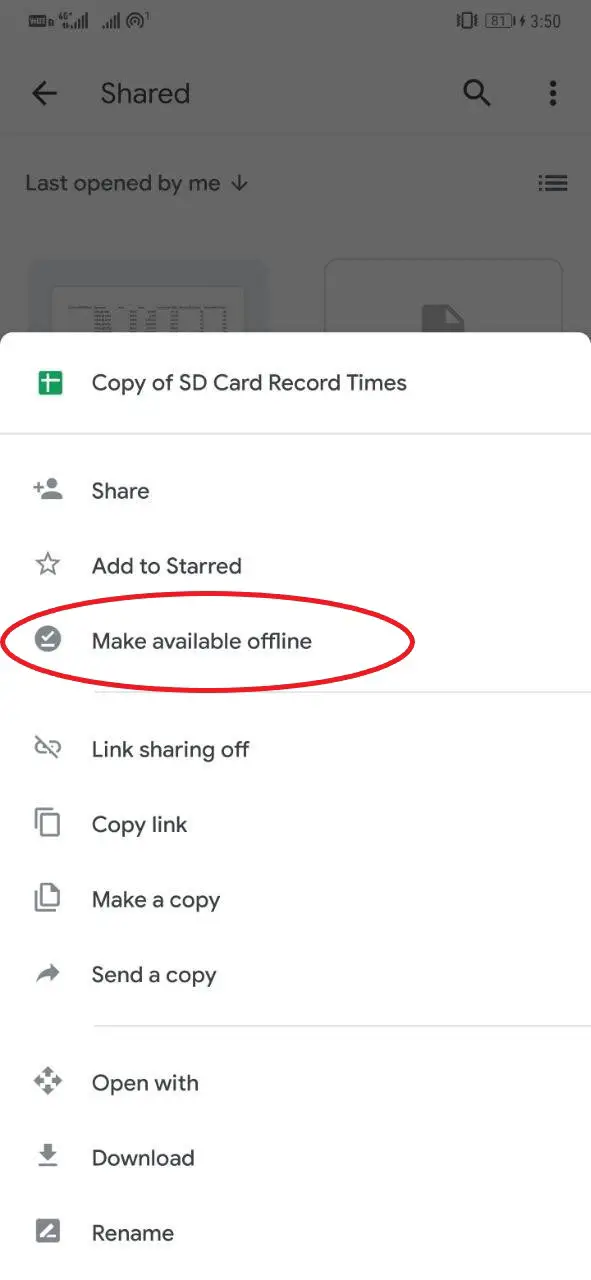Screenshot of the website options section. At the top, it displays the title "Copy of SD Card Record Times." The first option listed is "Share," followed by "Add to Start" and "Make Available Offline"; the latter option is highlighted with a red oval for emphasis. Additional options include "Link Sharing Off" and "Copy Link." The interface clearly aims to manage sharing and accessibility features for the file.